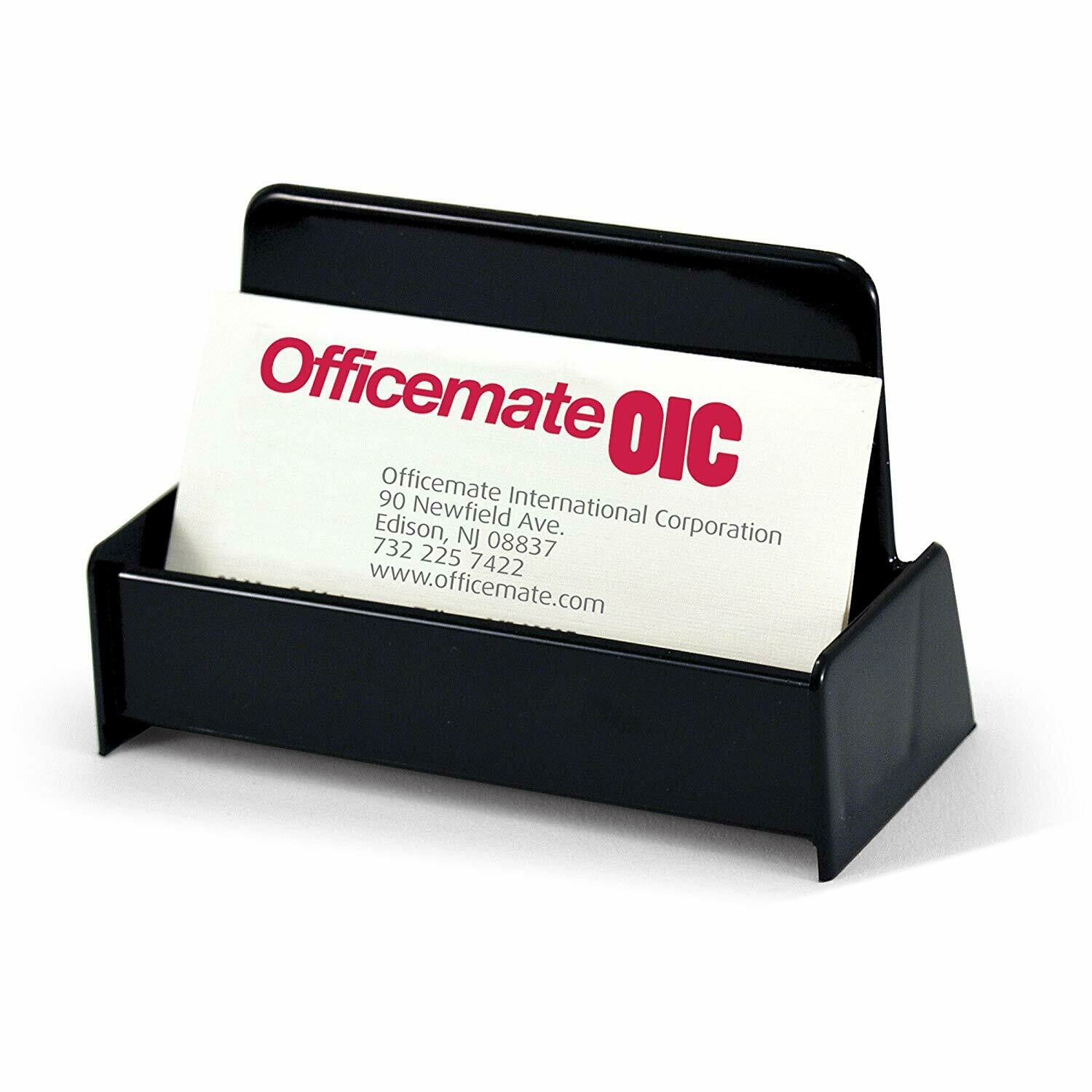The image shows a sleek black card holder positioned against a solid white background. The card holder, made of some type of plastic, features a rectangular base with raised edges, and the back is taller than the front, providing support for the card inside. The edges of the holder are slightly rounded at the top. Inside the holder, there's a single business card. The card is plain white and positioned in the center of the image, displaying text in bold and readable fonts. At the top, "OfficeMate" is written in prominent red letters, followed by "OIC" in capitalized red bubble letters to the right. Below this, the card provides detailed contact information: "OfficeMate International Corporation, 90 Newfield Ave, Edison, New Jersey, 08837-732-225-7422." At the bottom, the web address "www.officemate.com" is listed in black text. The overall color scheme of the image is black, white, and red, making the text stand out clearly, reminiscent of a potential office setting or product listing advertisement.